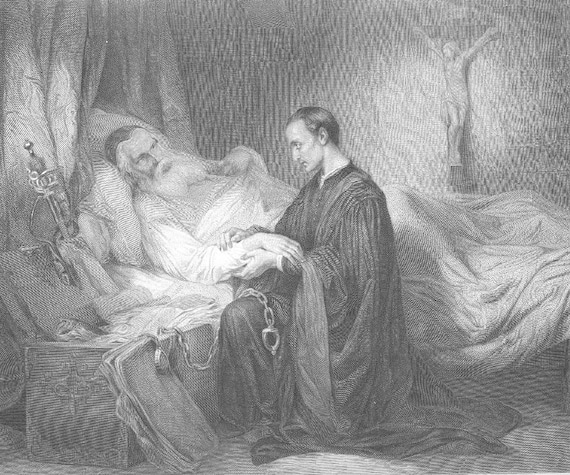The image is a finely rendered black-and-white sketch with no border or text. It features an older man lying on a low bed, partially covered by white sheets. The man, appearing gravely ill or dying, has white facial hair and still-visible darker hair on his head. He wears a white gown and a dark skullcap. His right arm is gently held by a kneeling man who appears to be a priest, dressed in a long black robe with buttons down the front. The priest, possibly in his 40s, has short dark hair and is looking down, his eyes seemingly closed in prayer or contemplation.

The scene’s background is detailed with vertical dashed lines forming the wall and curved dashed lines for the floor, giving the setting an almost tactile texture. On the wall hangs a slightly faded crucifix, showing Jesus with outstretched arms, nailed at the hands and feet, wearing a loincloth. A curtain drapes from the upper left corner, partially framing the scene.

Next to the bed on the lower left is a treasure chest, from which a chain drapes over the priest's right knee. The chest contains ornate items including a sword with an elaborate hilt. Additional small details, such as filigree and a cross-shaped decor on the chest, add to the richness of the composition. The image evokes a medieval or European style, capturing a poignant moment of solace and impending loss.